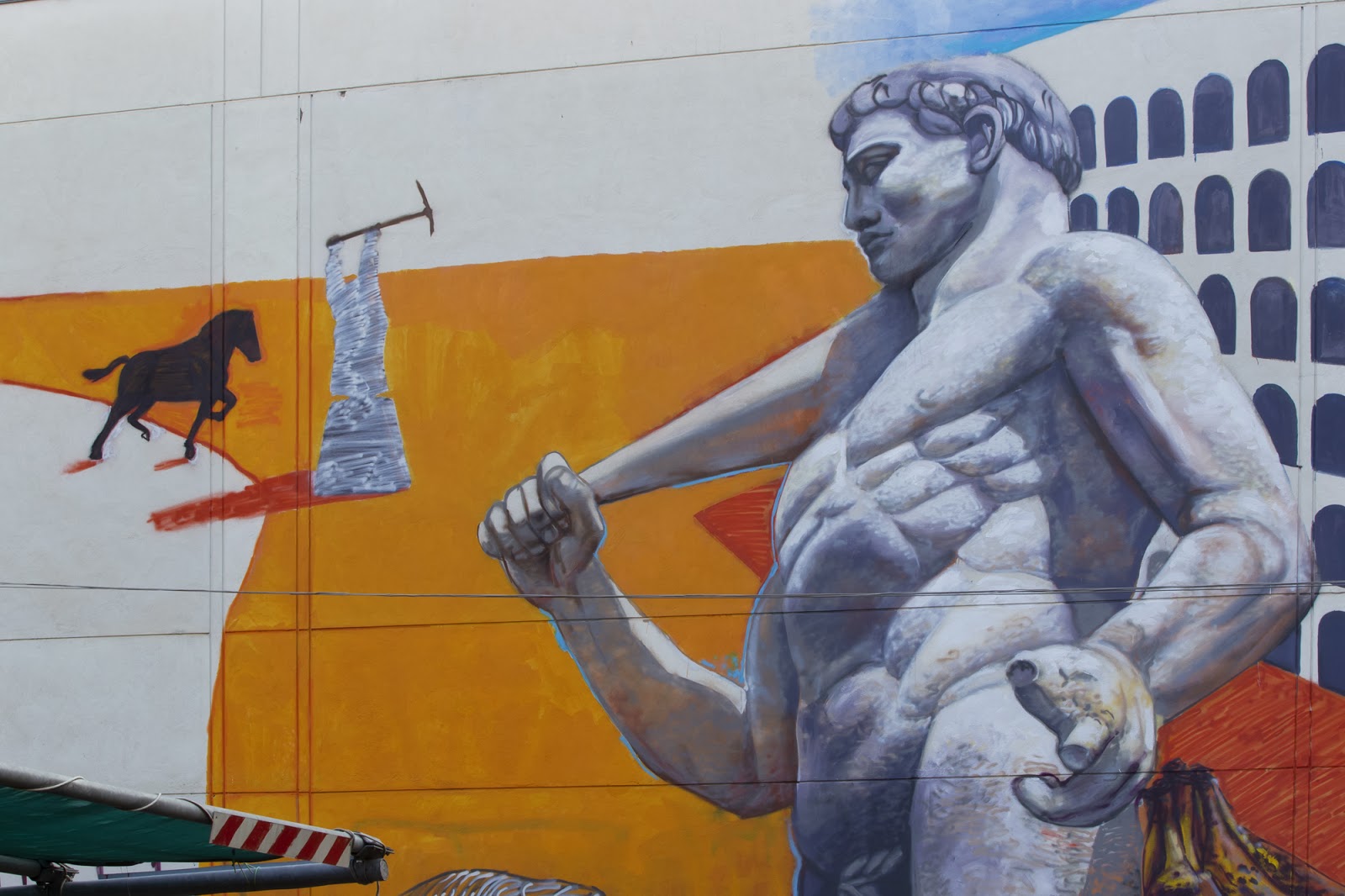The image is a detailed photograph of a horizontal rectangular mural, divided into various sized rectangles, primarily horizontally aligned. The upper left side of the mural transitions from a white background to light blue and then to sky blue towards the right. Below this transition, there's a simple white building with six rows of vertically aligned, arched black windows, partially obscured by a prominent white statue in the foreground. The statue features a muscular, nude male figure with a close-trimmed beard, wavy short hair, and a serious expression. He holds a tapered stick or bat on his left shoulder and his right hand is partially open but broken off. 

To the right of the statue is a stark orange background, which surrounds another white statue of a smaller person holding a pickaxe, casting a red shadow. The mural also features a silhouette of a horse behind the statue with red shadows around its lifted feet. Additionally, there is a narrow black triangle with diagonal orange and white stripes near the bottom left. The artwork is rendered in a mixture of colors including red, orange, gray, black, white, and light blue, and appears to possibly be a mural in Greece or Rome, with influences of classical and modern art styles.